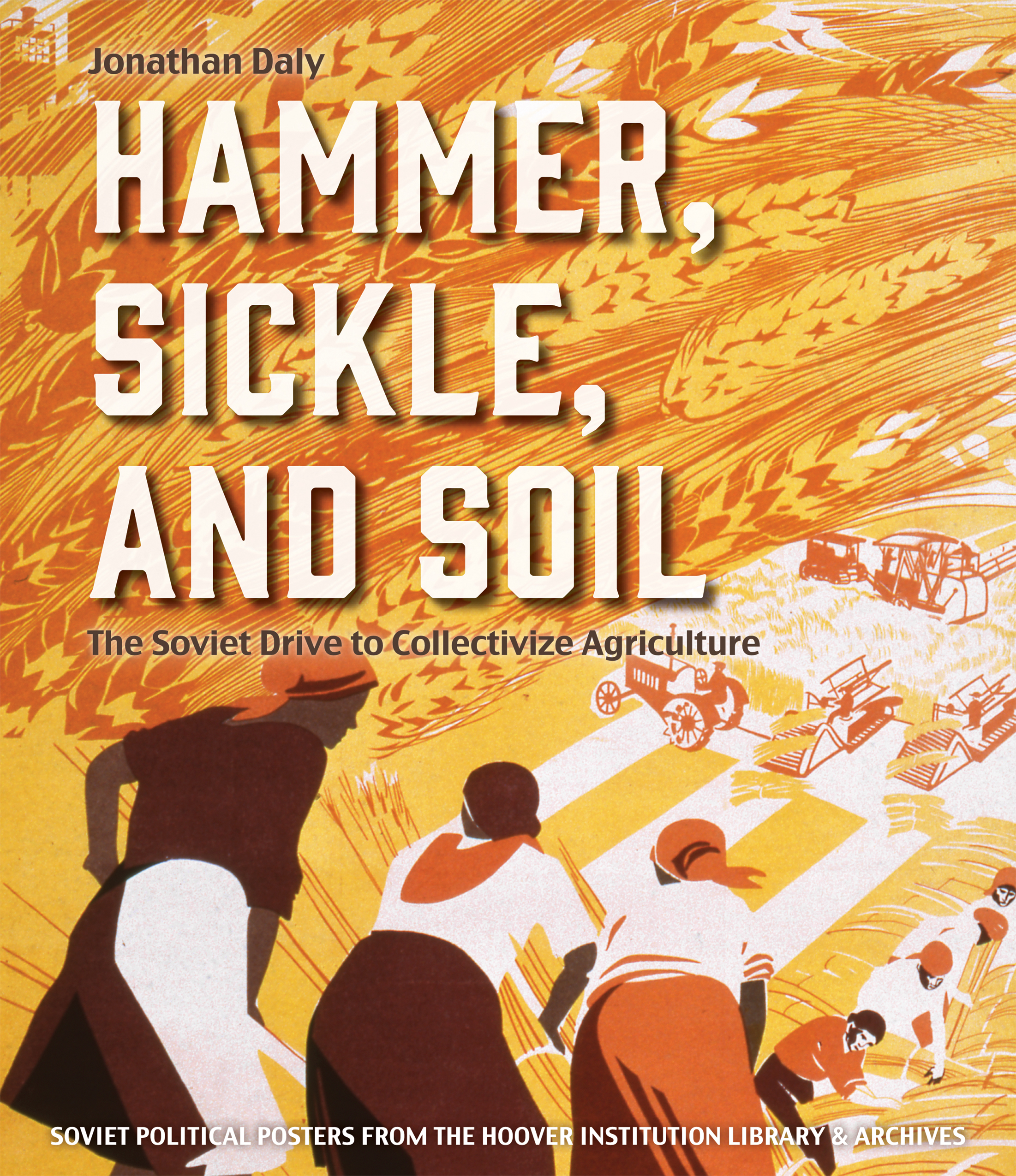The poster, titled "Jonathan Daly, Hammer, Sickle, and Soil: The Soviet Drive to Collectivize Culture," prominently features Soviet political posters from the Hoover Institution Library and Archives. It is a vivid computerized drawing with a palette dominated by yellows, golds, oranges, and whites. The background showcases rich tones of sheaves of wheat, symbolizing abundance and agricultural focus.

In the upper left corner, in bold black text, it reads "Jonathan Daly." Directly below, large white uppercase letters pronounce the title "Hammer, Sickle, and Soul," followed by "The Soviet Drive to Collectivize Agriculture" in darker lettering. The bottom segment of the poster, highlighted in white text, reiterates the source of the collection: "Soviet political posters from the Hoover Institution Library and Archives."

The artwork vividly depicts a bustling agricultural scene. At the bottom of the image, the foreground features three women, seen from behind, wearing skirts and head coverings, busily bundling wheat. To their right, men are actively involved in gathering the bundles. Additional figures, including agricultural men sowing and reaping, add to the dynamic portrayal of labor. Farming equipment is interspersed throughout, emphasizing the mechanized aspect of the Soviet agricultural drive. The upper left corner of the poster also includes a notable red design, enhancing its visual impact.